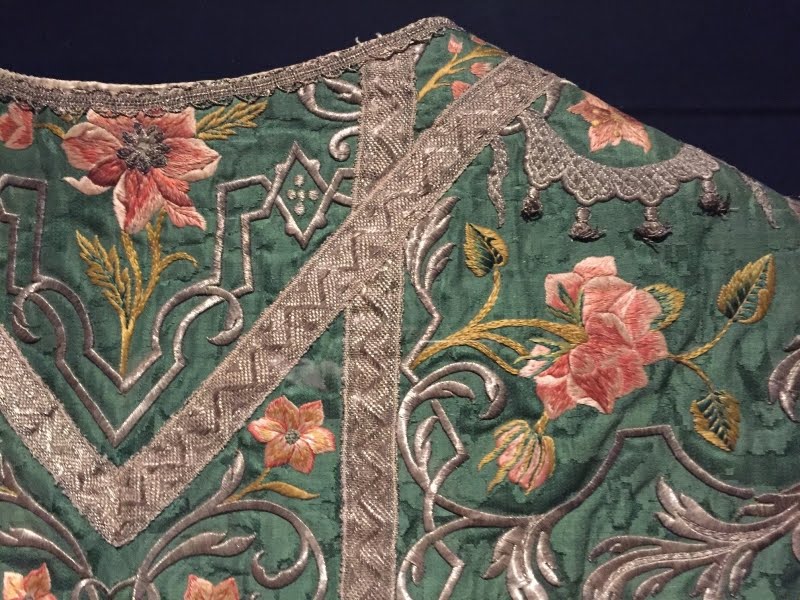This photograph features a close-up of a richly detailed, vintage green dress that appears slightly worn with age. The dress's deep forest green fabric is intricately embroidered with a floral pattern consisting of peach and pink flowers, accentuated by green stems and leaves, and further enhanced with delicate silver vines winding throughout. The neckline and collarbone region are adorned with silver borders and decorations arranged in a V-shape, with an additional vertical silver line extending downward, creating an ornamental and symmetrical design. Adding to its elaborate craftsmanship, the dress also features silver scroll designs that resemble leaves or feathers, as well as potentially crochet or felted elements, contributing to its unique and handmade look. Small metallic bells or baubles dangle from the shoulder area, offering subtle movement and a hint of a traditional or exotic origin. A lacy silver-gray material at the top gives it a delicately finished look. The background of the image is pure black, which contrasts starkly with the intricate details and colors of the dress, making them stand out prominently.